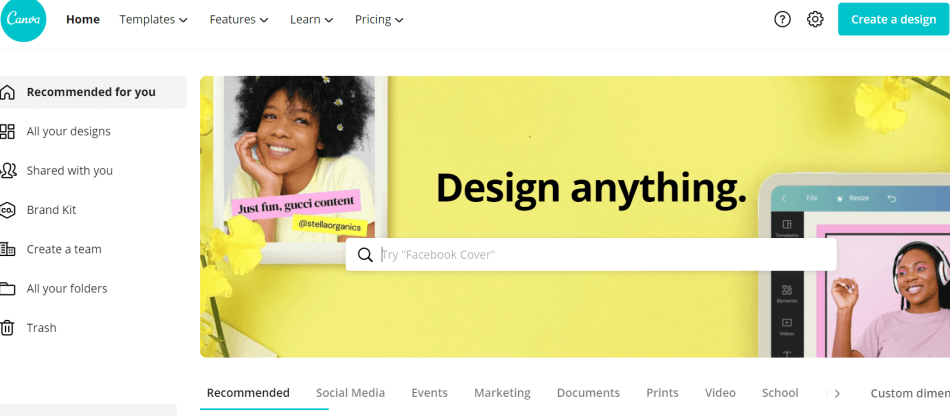Screenshot of the Canva Website Interface

The screenshot features the Canva website, a comprehensive online graphic design tool. Dominating the top-left corner, the distinctive Canva logo, a white script within a blue circle, is prominently displayed. Adjacent to the logo on the right is the main menu with options: Home, Templates, Features, Learn, Pricing, along with icons for Help (question mark) and Settings (gear icon). At the top-right corner, a light blue "Create a design" button stands out.

On the left side of the interface, there is a vertical menu bar featuring a series of icons and options: a house icon for "Home," a diamond icon for "Recommended for you," a grid icon for "All your designs," a two-person icon for "Shared with you," a palette for "Brand Kit," a group Icon for "Create a team," a folder icon for "All your folders," and a trash can for "Trash."

Towards the center-right of the screen, a vibrant yellow field showcases an image of an African-American woman with frizzy hair, posing thoughtfully with her hand under her chin. Behind her, the yellow background is adorned with flowers, giving the image a lively touch. A search bar above the image prompts users to "try Facebook cover." The phrase "Design anything" is boldly printed in black text over the yellow background.

At the bottom right of the screenshot, a smaller image displays a woman wearing headphones, likely illustrating design work in progress on a laptop or smartphone. Various category labels such as "Social media," "Events," "Marketing," "Documents," "Pricing," "Video," "School," and "Custom dimensions" are arranged along the lower part of the screen, highlighting the versatile design templates available through Canva.